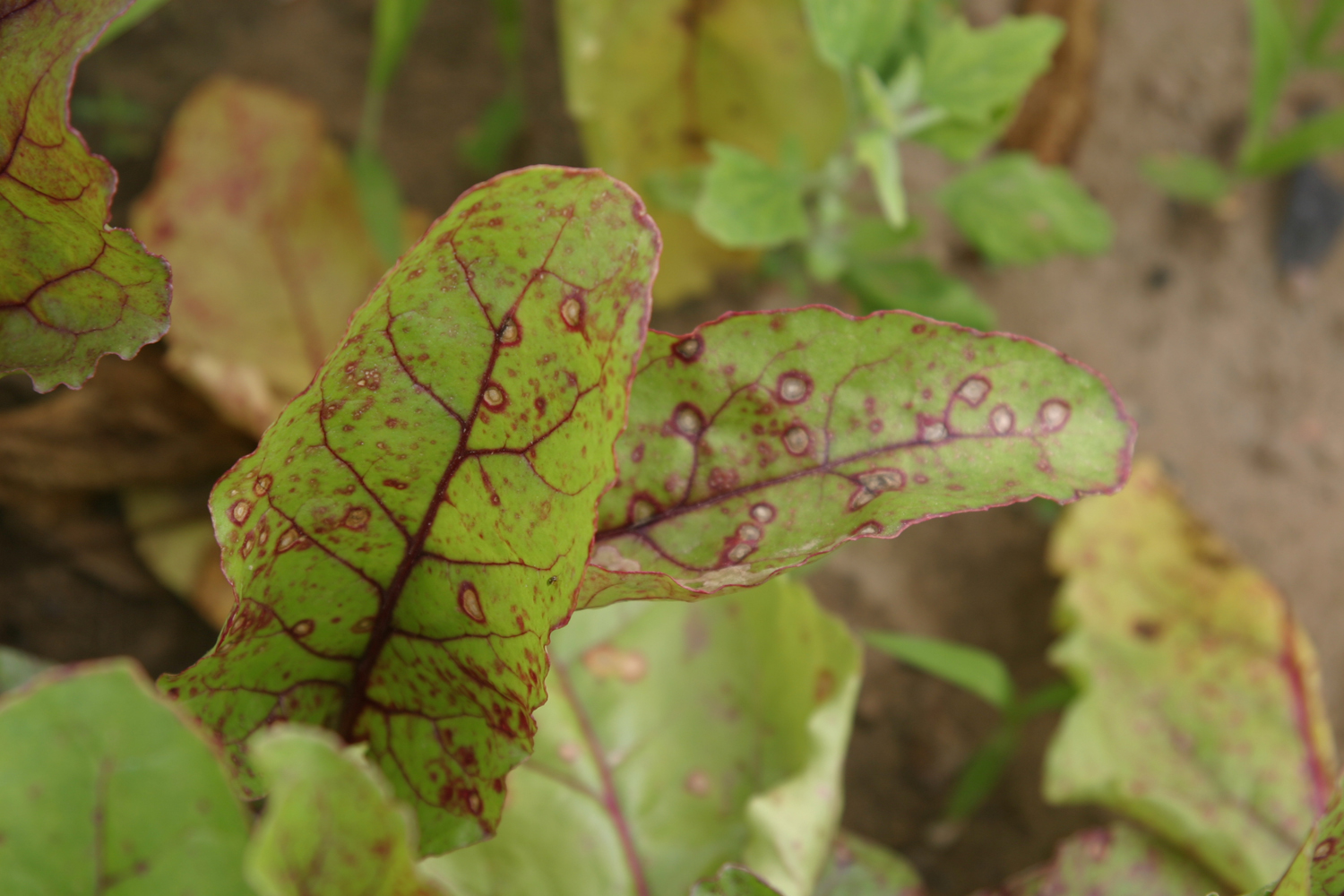The photograph captures a close-up view of foliage, focusing on two elongated, oval-shaped leaves in the center. These leaves, a bright green, are accentuated by prominent deep red veins running down their middles, which stand out starkly against the green. Both leaves exhibit signs of deterioration, visible through multiple red and white speckles and small holes, likely caused by insect activity. The leaf on the left shows a distinct bite mark along its edge. Surrounding these focal leaves, the background is noticeably out of focus, revealing a blur of brown and green hues, indicative of a dirt floor and additional indistinct leaves. A third leaf, positioned in the upper-left corner, is also partially in focus, echoing the detailed textures and damage seen on the central leaves.